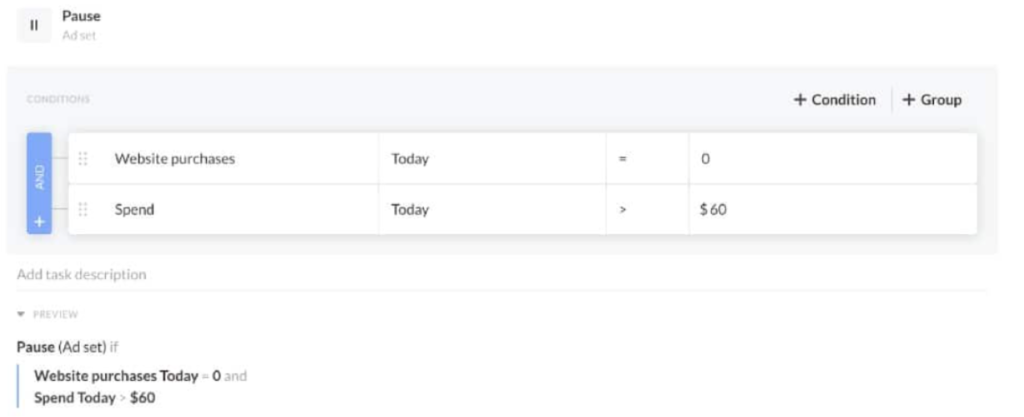This screenshot features a structured layout against a white background, divided into three distinct sections. 

The top section includes a small, light gray square housing two dark horizontal lines at its center. Adjacent to the square, the word "PAUSE" is prominently displayed in bold, black text, with "ADD SET" in a lighter gray text below.

The middle section is dominated by a long, light gray rectangle. Inside the rectangle, "CONDITIONS" is placed at the upper left corner in regular text. On the upper right corner, phrases "PLUS CONDITION" and "PLUS GROUP" appear in contrasting capital letters, with the latter in darker text. Within this rectangle, there is a table comprised of two rows and four columns.

The bottom third of the screenshot contains several textual elements: "ADD TASK DESCRIPTION," "PREVIEW," "PAUSE," and a conditional statement reading "SET IF WEBSITE PURCHASES TODAY EQUAL ZERO AND SPEND TODAY IS GREATER THAN $60."

This screenshot appears to be an interface for adding tasks or conditions, with a clear segmentation to guide the user through the process.